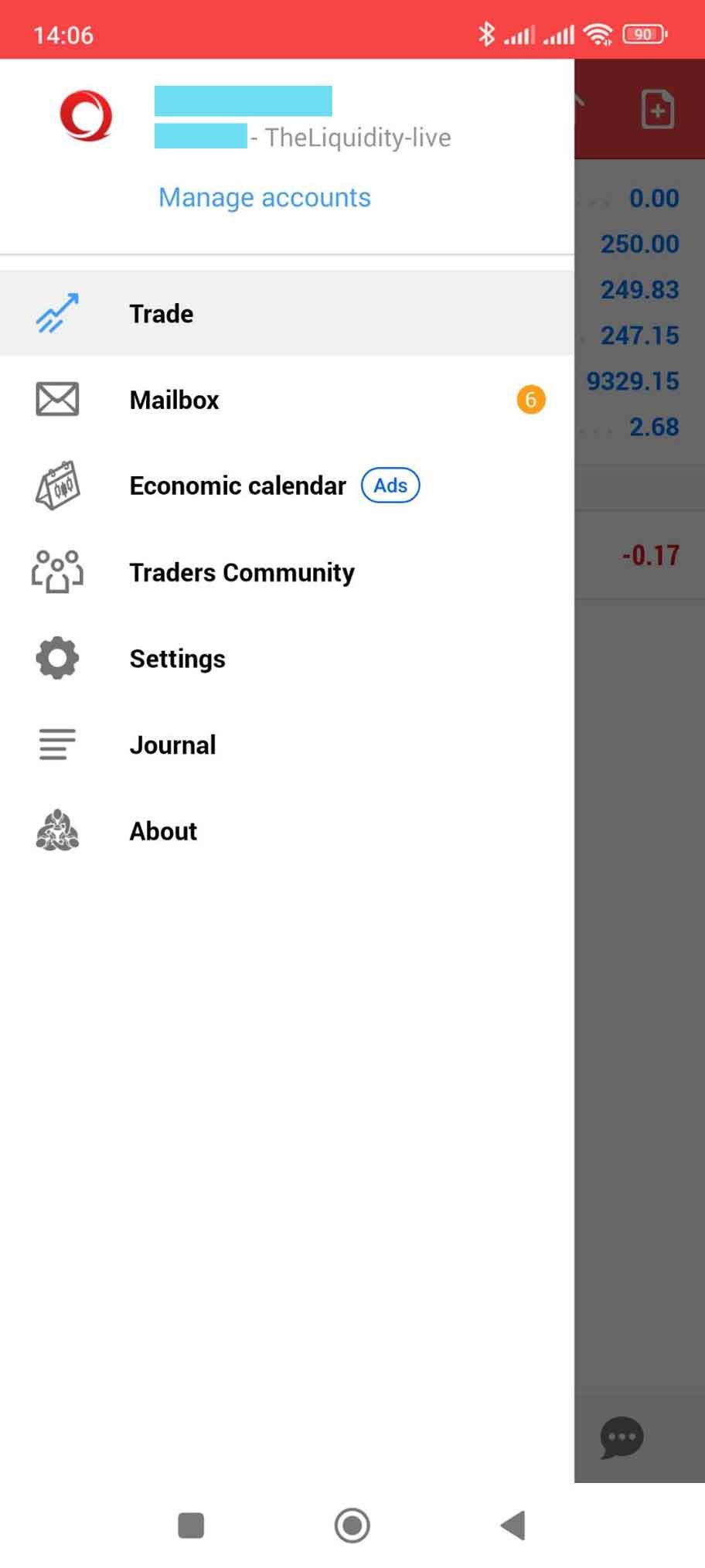This is a detailed caption for an image based on the provided voice description:

---

This image is a detailed screenshot from a mobile application. The status bar at the top clearly indicates this is a phone screenshot, displaying "14:06" on the top left corner, which suggests the time is 2:06 PM. On the top right, there is a battery icon, although the exact percentage is difficult to decipher due to blurriness; it appears to be either 96% or 80% charged.

Beneath the status bar, the main interface of the app is partially obscured, as a side menu has been pulled out from the left side of the screen. The background of the app is quite dark, making the brightly lit side menu the focal point of the screenshot. At the top left of the side menu, there is a small red circle and an area obscured with blue lines, possibly indicating the user's profile picture and name, which have been blurred for privacy.

Directly below these, the side menu lists various options: "Manage Accounts," "Trade Mailbox," "Economic Calendar," "Traders Community," "Settings," "Journal," and "About." This suggests that the user has opened a profile or settings menu within an app related to trading or financial management. At the very bottom of the screen, the familiar navigation buttons typical on smartphones are visible, with the home button centered.